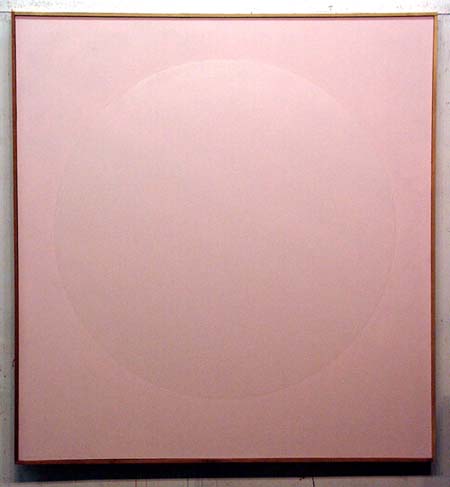This image captures a minimalistic and abstract artwork that is slightly taller than it is wide, exhibiting a rosy mauve pinkish square or rectangular center framed by a light brown or whitish-gray border. The border includes a distinct, thicker black line at the bottom edge. The center pink area contains a subtle circular imprint, as if a circular shape was pressed into the material, creating a visible, yet understated, mark. The artwork appears to be mounted on a concrete or white slab background, though only a small portion of the background is visible. No other elements or distractions are present in this composition, emphasizing the simplicity and abstract nature of the piece.